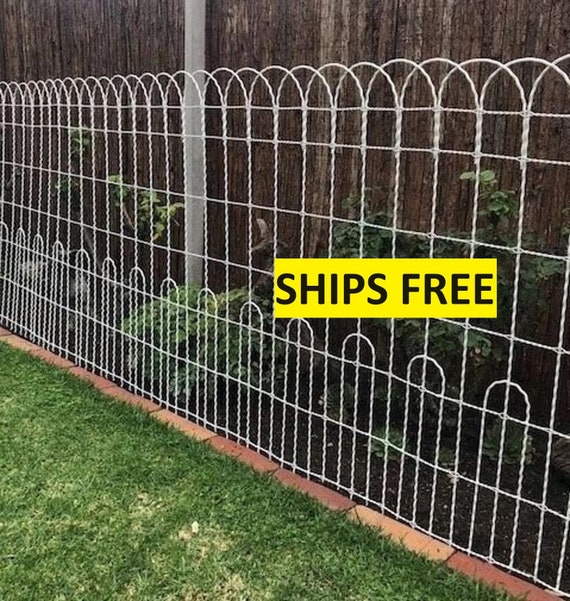The photograph captures a picturesque backyard scene featuring a small, fenced-in garden area. The most prominent elements are the two fences: an old, worn, and knotted brown wooden fence in the background and a delicate, white wire fence in the foreground. The white wire fence, designed with shapely, rounded grids and arching thin posts, stands firmly on a line of bricks that separates it from a lush, green lawn extending out of the frame. Between the wooden fence and the white wire fence, small plants fill the space, suggesting a protected garden or plant bed likely shielded from deer, rabbits, and other animals. In the middle-right of the image, a bright yellow block with the text "Ships Free" is conspicuously placed, possibly suggesting a promotional message for the white wire fence, though it appears out of context within this serene backyard setting.